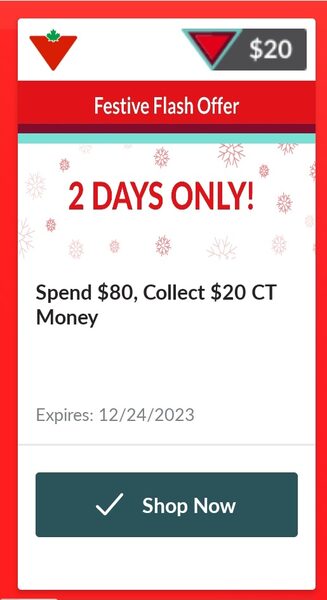This image features a festive flash offer prominently displayed in a portrait-oriented white box on a vibrant red background. The top left corner of the box showcases an upside-down triangle with a green leaf centered at the bottom portion of the triangle. On the opposite side, there is another upside-down triangle, this one red with a black outline and a secondary outline in a minty blue. Adjacent to this triangle, within a small gray box with white font, is the text "$20."

Directly below, a red banner features the phrase "Festive Flash Offer" in bold white font. Following this, a message in red font declares "Two Days Only!" accompanied by red snowflake icons. The central message, written in bold black font, reads "Spend $80, collect $20 CT Money." Just beneath this, the expiration date "Expires 12-24-2023" is stated in gray font.

At the very bottom, there is a dark blue box with white font that includes a check mark and the option to "Shop Now." The overall design clearly conveys the limited-time promotional offer, emblazoned with festive elements and clear calls to action.